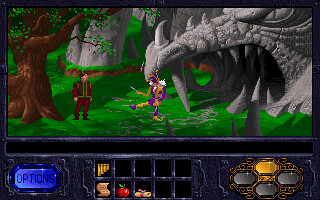This image appears to be a screenshot from a vintage video game, potentially dating back to the late 1980s or early 1990s. The scene exudes a distinct fantasy atmosphere, filled with intriguing elements. On the right side of the image, there is a cave ominously shaped like a dragon's head, with its mouth agape, displaying sharp teeth and a dark interior. The dragon's eye adds to the menacing aura of the cave. To the left, a grand tree towers over the landscape, adding a touch of nature to the fantastical setting.

In the middle of the scene stands two characters. The figure on the left is a man dressed in a red shirt and pants, adorned with a vest. He appears to be gazing towards the second character at the center, who is dressed in a colorful, jester-like outfit consisting of yellow and purple garments, topped with a white puff. The setting appears to be a lush, forested area, with visible grass underfoot.

The user interface (UI) of the game is also visible. On the bottom left of the screen, there's a blue button labeled "Options." In the center, a series of black squares display various items, including a yellow pan flute, a piece of parchment, an apple, and a scroll. On the bottom right, there are four oval indicators; the top one is gold, while the others are gray. This detailed depiction highlights the charm and complexity of early video game designs.